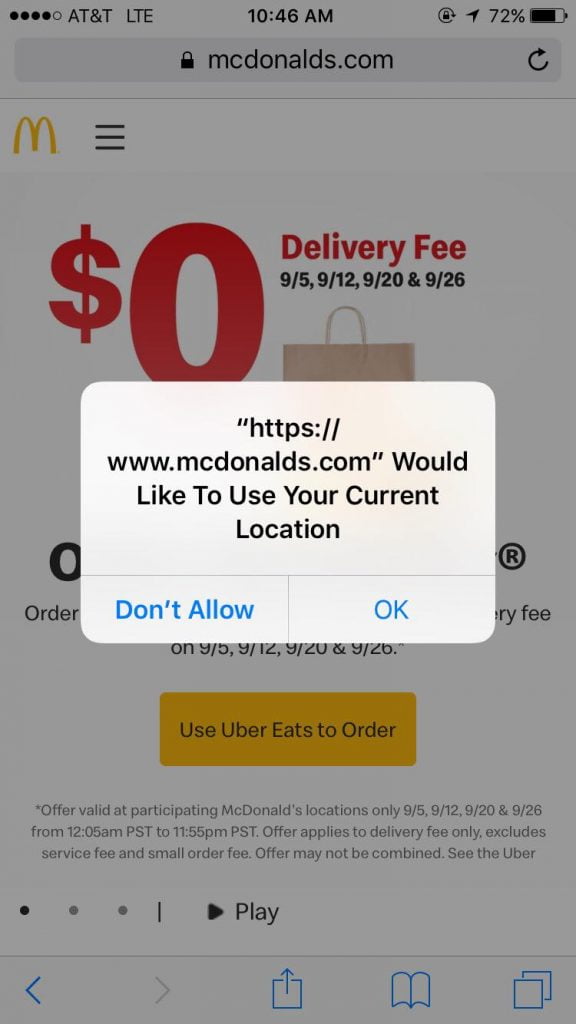The image depicts a McDonald's website viewed on a mobile phone screen. At the top left corner, the status bar shows AT&T with LTE connectivity. The time displayed in the center reads 10:46 AM, while the right side of the status bar shows two icons, one of which indicates the battery life at 72%.

Below the status bar, the browser's URL area displays "mcdonalds.com" with a yellow McDonald's 'M' logo to the left and a three-line tab menu icon. A red banner underneath promotes a "$0 delivery fee" for specific dates: 9-5, 9-12, 9-20, and 9-26.

The top part of a light brown paper bag is visible, followed by a pop-up message in the center of the screen stating, "mcdonalds.com would like to use your current location." The message provides two user options: "Don't allow" on the left and "OK" on the right, both written in blue text.

Further down, the message obscures part of the order status section. A yellow banner below encourages users to "Use Uber Eats to order," followed by an offer validity statement with additional small text. At the bottom, there's a play icon on the left and a blue arrow on the bottom left corner. The center features a share icon, followed by an open book icon and two overlapping blue squares to the right.